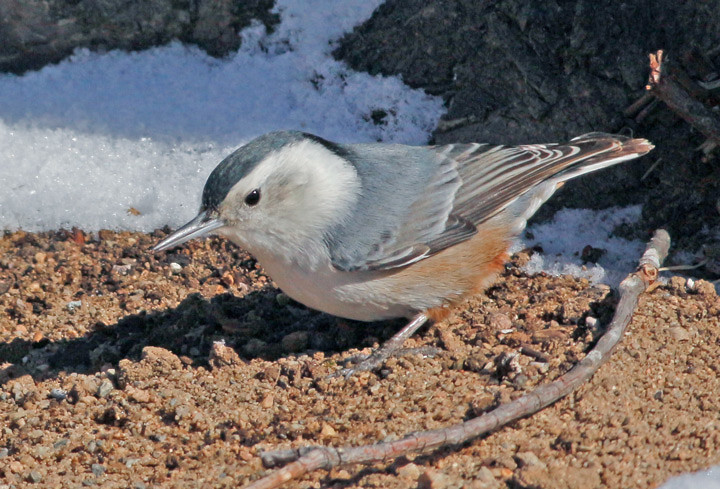The image is a landscape-oriented close-up photograph of a small bird, resembling a sparrow, standing on brown soil. In the background, there are dark gray rocks or the base of a mountain, with patches of snow tucked into the crevices. The bird is primarily gray with black and brown accents. It has a white face with a distinctive gray line that forms a big white cheek, and a short, pointy gray beak. The top of its head, back, and wings are medium gray with tinges of brown along the edges of the wing feathers. The chest area is white, while the area around the legs and the underside shows a reddish-brown hue. The bird's eyes are tiny and black, giving it a somewhat frowning expression. Its wings are held closely to its body, and it has a short tail. A brown stick with white knobs lies on the ground in front of it.